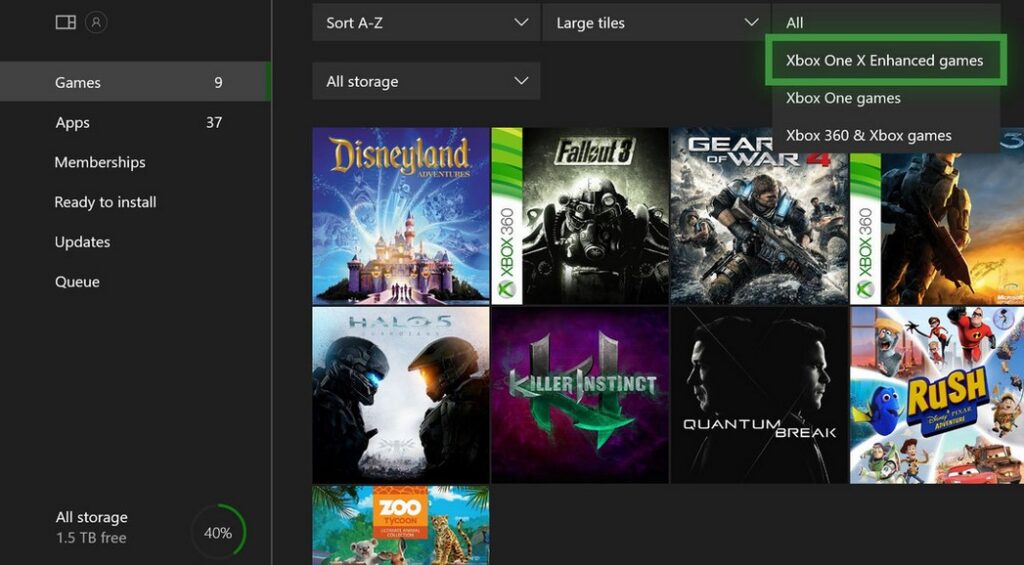This image is a screenshot showcasing an Xbox game menu. The interface features a very dark grey and black background, with a navigation column on the left-hand side. In the top left corner, there's an illustration of an old-style TV, depicted as a line drawing with a rectangle, a square, and two smaller squares. Below this, you'll find various navigation options. The current selection, highlighted against a dark grey background (distinct from the black), is for games, showing 9 results. Other navigation options include apps (37 results), memberships, ready to install, updates, and queue. 

At the bottom of the navigation column, it indicates the storage status with "all storage, 1.5TB free" and shows a usage graphic with a small green semicircle representing 40% used. The main content area of the screen, predominantly black, displays sorting options at the top in grey boxes: "Sort A to Z" with a dropdown, and "Large files" with another dropdown. The dropdown is opened, showing options like "Xbox One X enhanced games," "Xbox One games," "Xbox 360 and Xbox games," with "Xbox One X enhanced games" outlined in dark green. 

Beneath these options are 9 game thumbnails arranged in three rows: the top two rows containing four thumbnails each and the third row featuring a single thumbnail on the left-hand side.